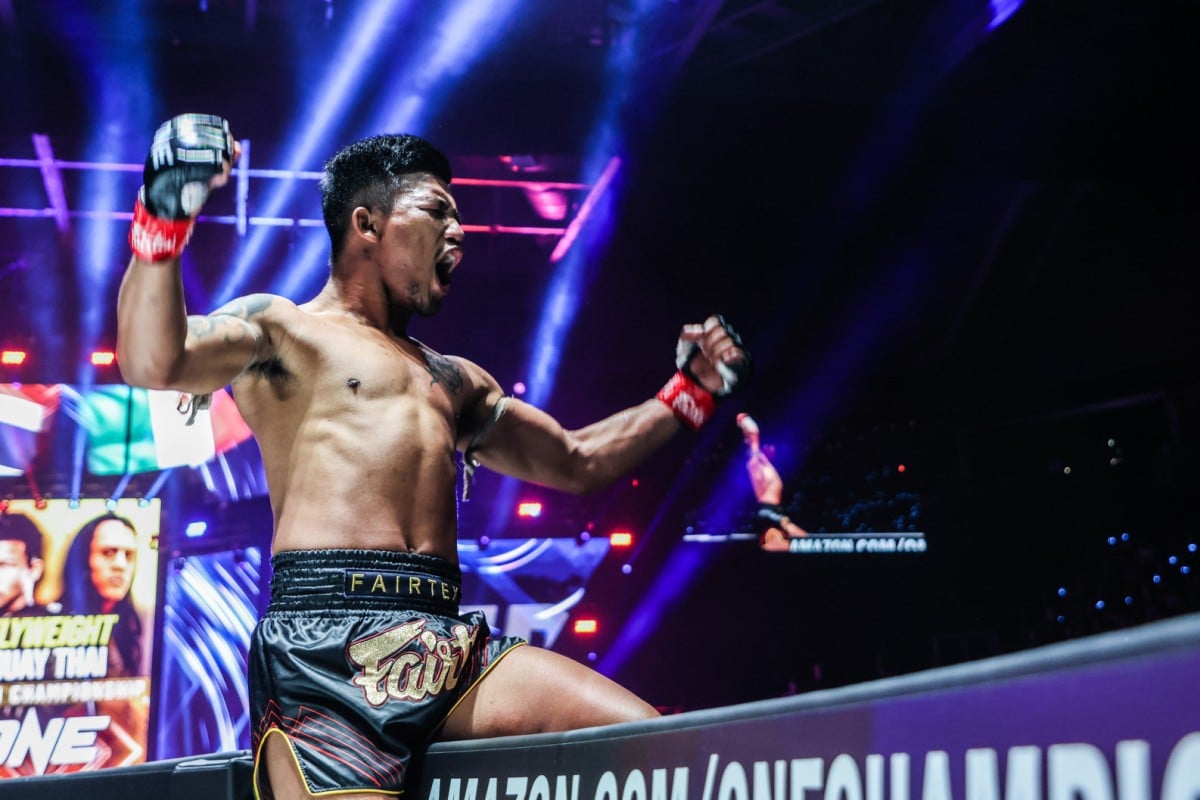The photograph captures Rod Tang, a renowned Muay Thai fighter, in an exuberant celebratory pose. He is straddling a sign or divider, raising both of his arms above shoulder height, hands clenched in black gloves with red straps. His expression is intense, mouth open as if yelling in triumph. Rod Tang, shirtless with short, dark hair styled into a buzz cut with the sides shaved, showcases a tattoo on his left shoulder and right arm. His fight shorts, colored black with accents of purple and yellow, prominently display the brand "Fairtex". Behind him, big screens and neon signs project fight posters and images that add to the atmosphere of a festive and energetic sporting event. The scene suggests that he has either just finished a victorious fight or is preparing for one, exuding confidence and strength.